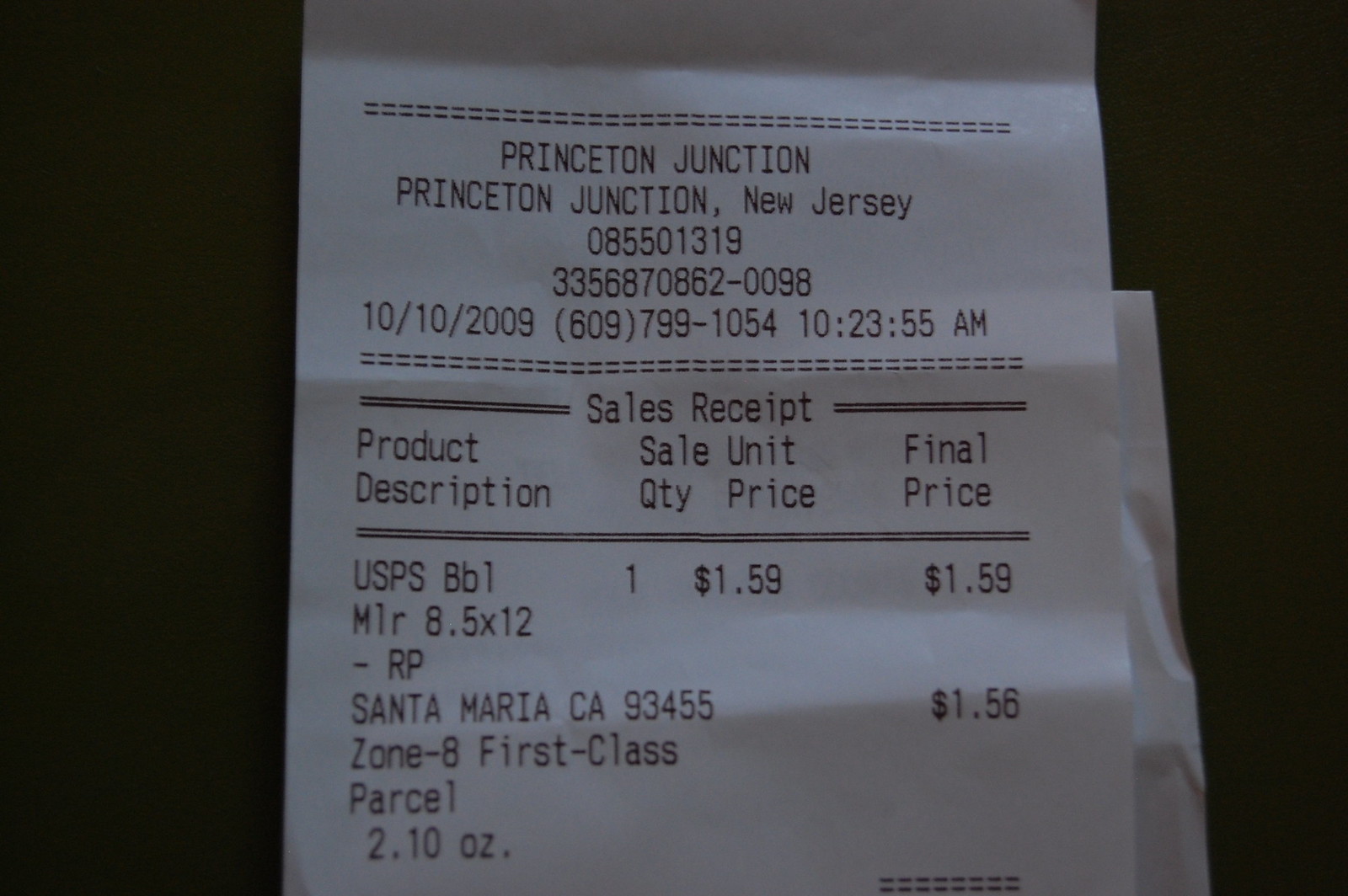This photograph captures a detailed image of a receipt from Princeton Junction, a location in New Jersey. Dated October 10, 2009, the receipt includes the phone number and exact time of printing. The top section prominently labels it as a sales receipt, followed by columns detailing product descriptions, sale units, quantities, prices, and final totals. The primary item purchased is a USPS BBL, costing $1.59. 

Additionally, the receipt lists dimensions of 8.5 by 12 inches, indicative of shipping details. It mentions another location, Santa Maria, California, 93455, possibly the destination of the parcel, with an associated cost of $1.56 likely representing shipping charges. This transaction is noted to be for a first-class parcel delivery weighing 2.1 ounces, information found near the bottom of the receipt.